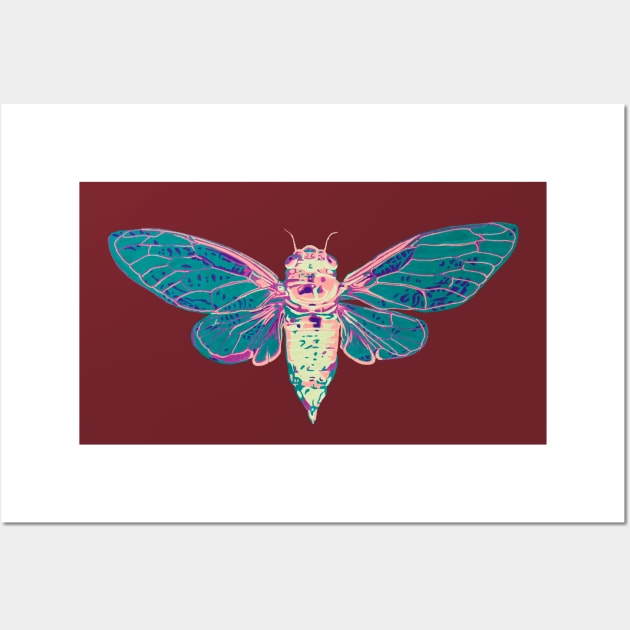The image appears to be an illustration of a butterfly, centered within a horizontal rectangular frame that sits on a square gray background. The butterfly is depicted from a top-down perspective, revealing its eyes, body, and spread wings. The primary body of the butterfly is adorned in golden, pink, and a hint of aqua colors, tapering to a point at the back. The wings are predominantly aqua, with the front and back edges accented by pink. The butterfly's antennae, which are also pink, extend gracefully from its head.

Enclosing the butterfly illustration is a dark red background, bordered by white matting or wire, giving the image a polished, clean appearance. The framing further accentuates the vibrant colors of the butterfly, creating a striking visual contrast. This intricate and detailed depiction effectively captures the elegance and delicate structure of the butterfly, devoid of any visible legs, adding to its ethereal quality.